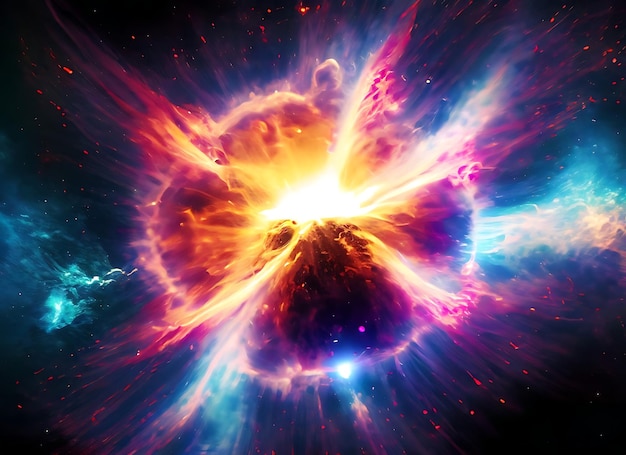This vibrant, futuristic image appears to be a digital artwork, possibly created through computer graphics. The composition is a wide rectangle, predominantly featuring a dramatic explosion in the center against a mostly black background. The explosion, evocative of a sci-fi or outer space theme, is predominantly white and yellow at its core, radiating outwards with a dazzling array of colors. Bright oranges, hot pinks, and various shades of red give the central explosion an intense, fiery quality, with colors transitioning into purples and blues as they spill outward from the center. 

On the left side, a blue, cloudy-looking section contrasts the explosive core, which is surrounded by darker tones in the four corners of the image. The explosion seems to extend outwards with large, vivid plumes and squiggly blue tendrils, while numerous small red speckles, reminiscent of glowing embers, are scattered throughout the darker areas, adding to the dynamic and energetic feel of the piece. The overall effect is both spectacular and surreal, making it look more like a stunning piece of sci-fi art than anything found in real life.